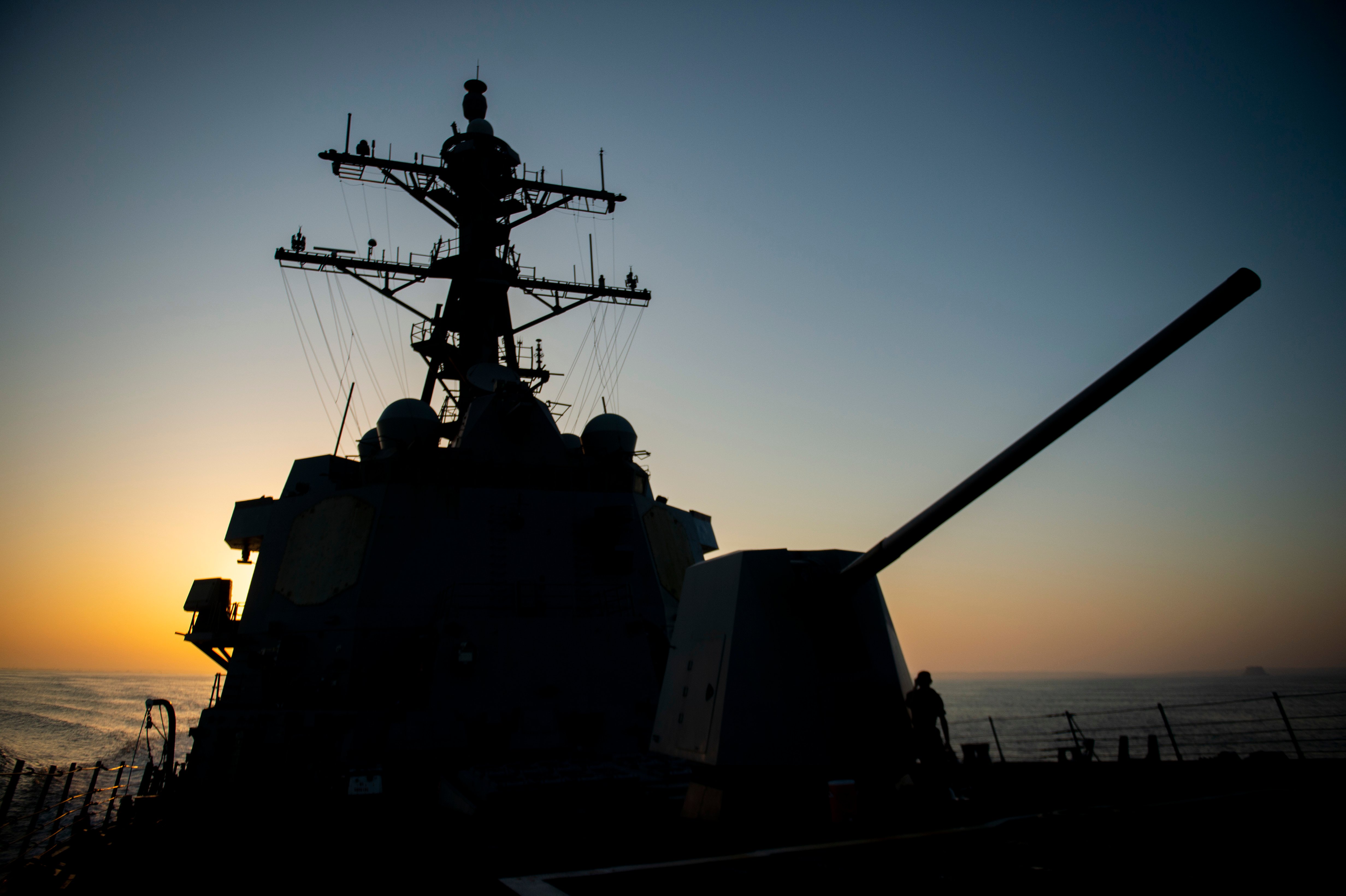In an evocative silhouette during what seems to be either dusk or dawn, a battleship stands against a gradient sky that transitions from light blue to dark. The horizon is tinged with a golden-yellow glow, indicative of the sun either setting or rising. The photograph appears to be taken from the deck, focusing on the tower-like section of the ship adorned with radar arms reaching skyward. A large caliber gun juts prominently to the right, its imposing form silhouetted starkly against the backdrop. Below the gun, a lone person is kneeling, their figure just a shadowy outline. At the edge of the deck, a cloth fencing is visible, possibly serving as a safety measure to prevent falling overboard. The entire scene is rendered in deep, dramatic shadows due to the low light source that casts the ship into near darkness, leaving the details enveloped in mystery and intrigue.